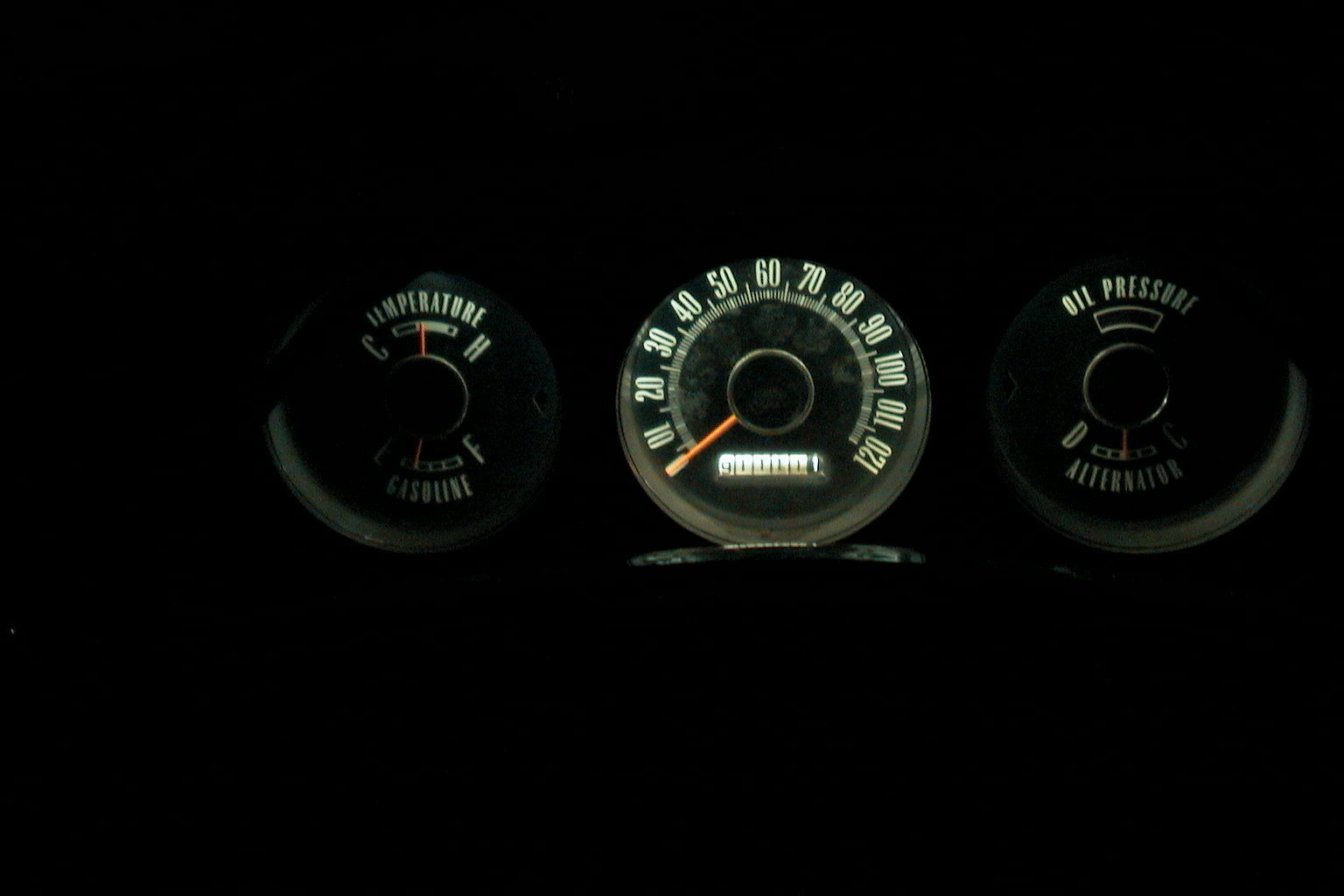This photograph, taken inside a dark space, captures the illuminated dashboard dials of a vehicle. The image prominently features three circular gauges:

1. **Top Left Dial**: This gauge displays temperature with a bar indicating 'C' for cold and 'H' for hot, and a red needle hovering in the middle. Below the temperature indicator is a gasoline gauge, with 'E' for empty and 'F' for full; the red needle shows the tank is one-quarter full.

2. **Center Dial**: This central dial is a speedometer reading from 0 to 120, with the needle resting at 0. Below the speedometer, there are additional smaller dials with incremental numbers, though the details are unclear.

3. **Top Right Dial**: Labeled "Oil Pressure," this gauge has an empty black bar below, and beneath it, another gauge marked "Alternator." The alternator indicator shows 'D' and 'C' with a red needle positioned in the middle of the bar.

This detailed portrayal highlights the critical vehicle metrics, visible due to the soft glow from the dashboard lights against the dark backdrop.